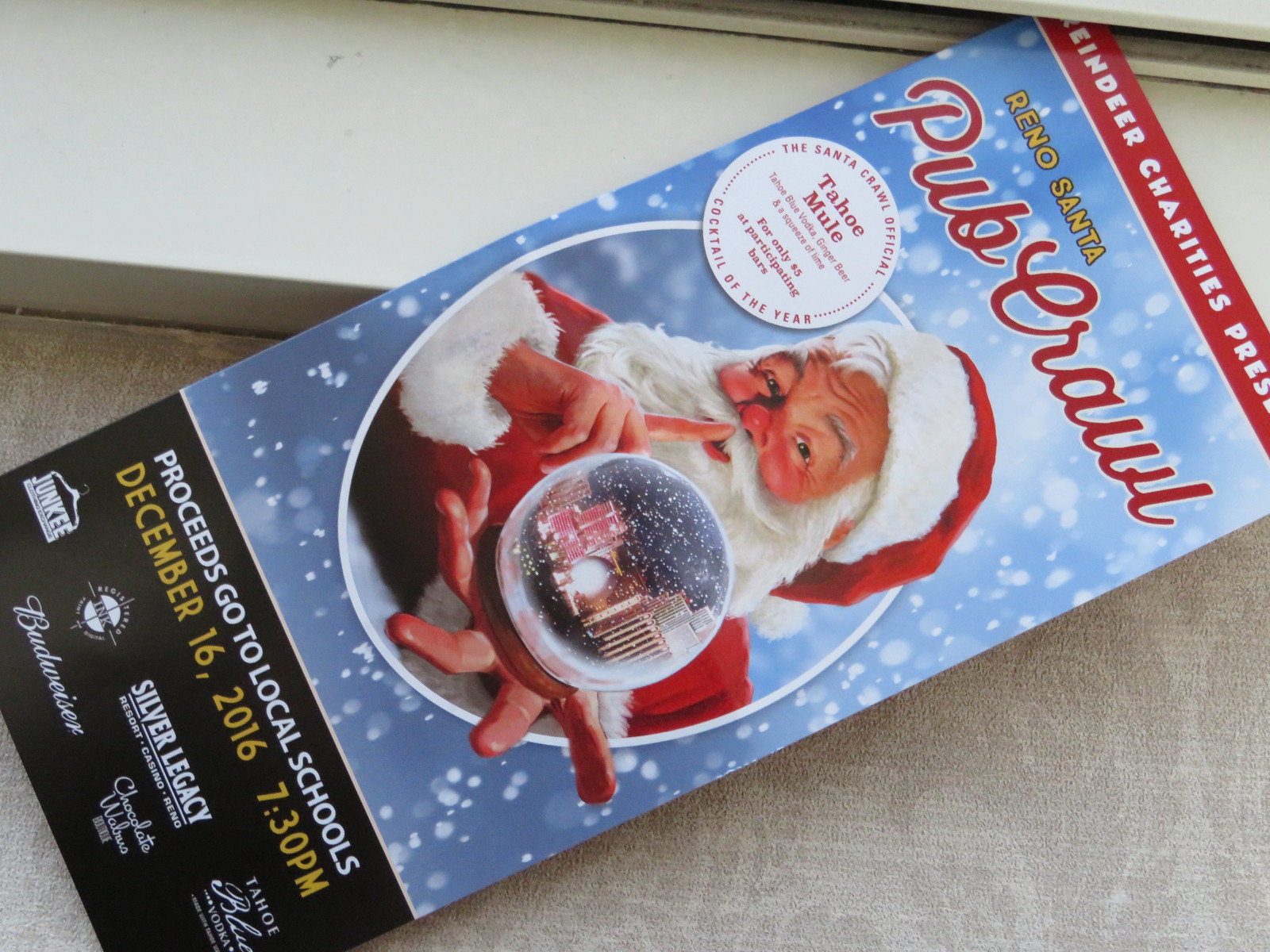The image is a close-up photograph of a Christmas event flyer, leaning diagonally against a window ledge. The flyer prominently features a graphic of Santa Claus in the center, wearing his traditional Santa suit and holding a snow globe. Santa has his right finger pressed to his lips, signaling a secretive "shh." The background of the flyer is predominantly blue, resembling a snow globe, with a red banner across the top. The banner reads "Reindeer Charities Presents" and below it, "Reno Santa Pub Crawl." 

In the middle portion, there is an announcement in red letters about the event featuring the Tahoe Mule cocktail, made with Tahoe Blue Vodka, ginger beer, and a squeeze of lime, available for $5 at participating bars. Towards the bottom of the flyer, a black rectangular banner states that proceeds will benefit local schools, with event details specifying December 16, 2016, at 7:30 p.m. Additionally, several sponsors are listed at the bottom, including Budweiser, Silver Legacy Resort Casino, Junkie, Chocolate Walrus Boutique, and Tahoe Blue Vodka. The whole flyer is colorfully detailed with red, blue, and black elements, folded at an angle, contributing to an organized yet festive composition.